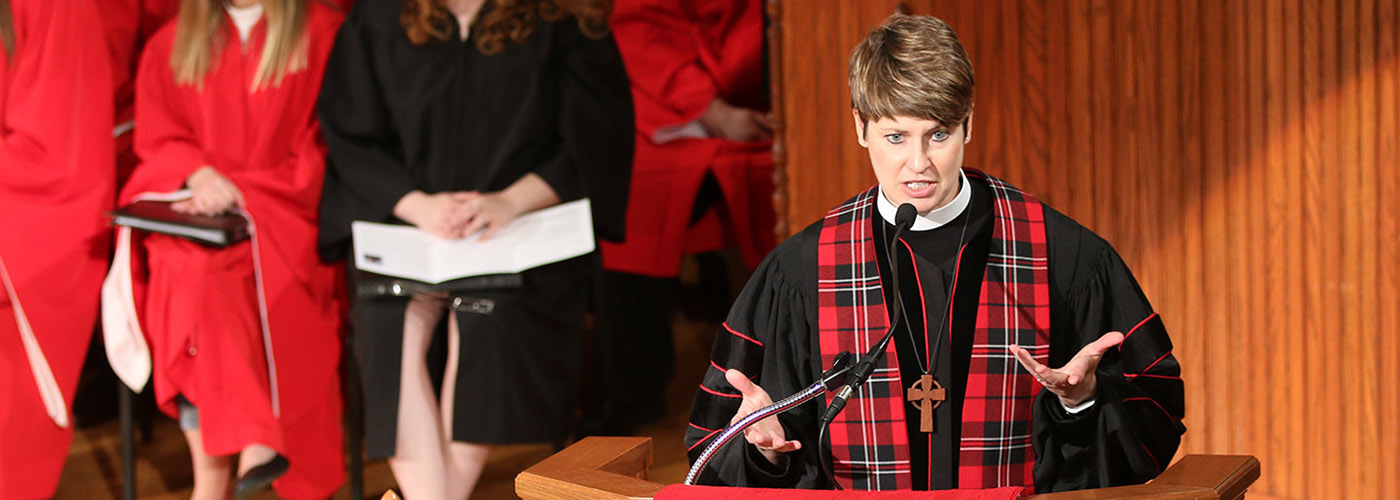The photograph captures a woman in a black robe, speaking passionately from a wooden podium positioned to the right of the center of the image. She has short brown hair and is adorned with a red checkered scarf around her neck and a brown wooden cross necklace. The details of her attire and accessories hint that she might be a pastor or deacon, and she gestures expressively with her hands during her speech. The setting is well-lit and clear, with several women seated on the left side of the image. These women, dressed in either red or black robes, hold books—some open to show white pages and others closed with black covers. The scene appears formal, possibly within a church or academic environment, suggested by the wooden platform and the wooden panel finishing in the background. The audience members' attire and presence of books suggest a ceremonial occasion, such as a graduation or a religious service.